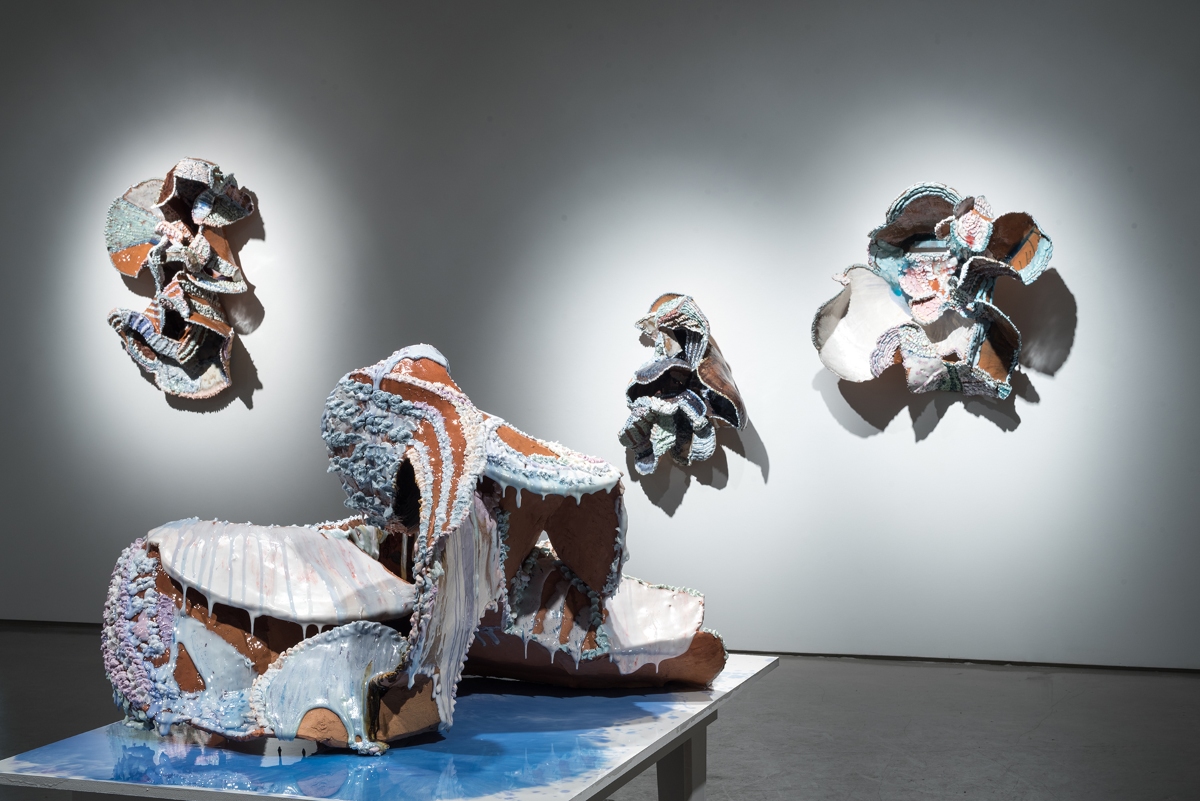The image features an art installation in an art gallery, characterized by a gray floor and white walls. Central to the composition is a low table with a blue marbled top, located towards the lower left. Atop this table sits an abstract sculpture, predominantly brown with elements of white, blue, and purple. The sculpture resembles a crumpled form with sections that appear like bent cardboard, enhanced by dripping paint on its edges. Surrounding this centerpiece are three additional abstract pieces, mounted on the wall behind the table. These wall-hung sculptures share the crumpled appearance and irregular shapes of the primary piece, with lights strategically illuminating each one to emphasize their textural details and color variations. The overall arrangement and focused lighting further underscore the gallery setting, enhancing the modern and abstract nature of the art installation.